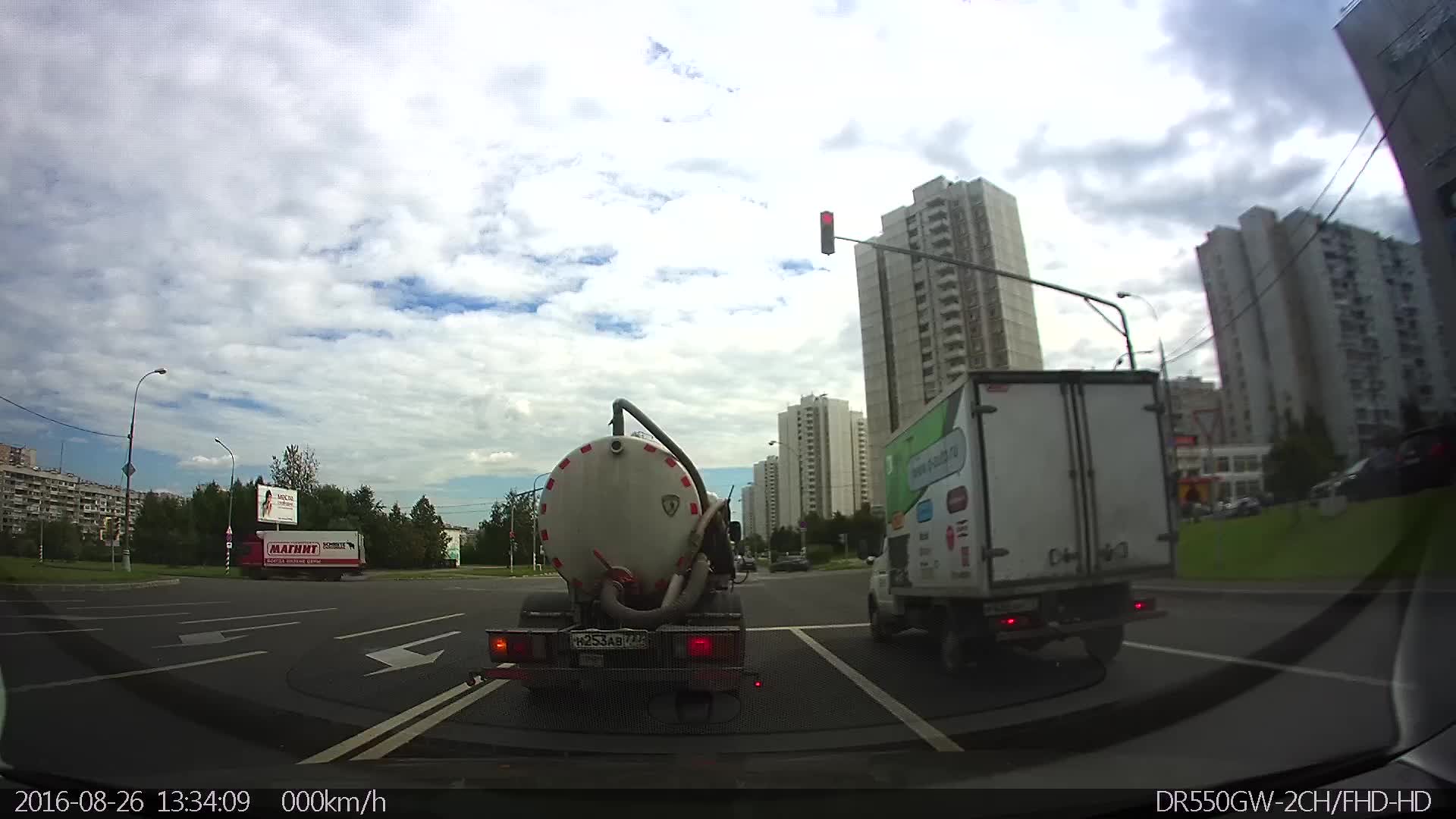This photograph, captured from a police camera on August 26, 2016, depicts a bustling city streetscape viewed through the windshield of a stationary vehicle. The vehicle, stopped at a red light, faces a large oil tanker truck directly ahead. To the right of the tanker is a medium-sized delivery van, identifiable by its white cab. Both trucks have their red tail lights illuminated, emphasizing the stoplight's red signal. The street comprises four lanes, with two trucks occupying the nearest lanes. In the far lane, a truck is visible, turning left at the intersection, aligning with a small billboard to the left.

Prominent in the scene are various buildings: a tall apartment complex stands before the second vehicle in the far lane, while shorter buildings flank the street on either side. The sky above is predominantly cloudy with occasional patches of blue, adding a dynamic backdrop to the urban environment. Sprinkled around are instances of greenery and modern street infrastructure, including a streetlight that arches over the roadway and the conspicuous stoplight governing the intersection. Overall, the image provides a detailed view of city life captured in a moment of pause at the intersection.